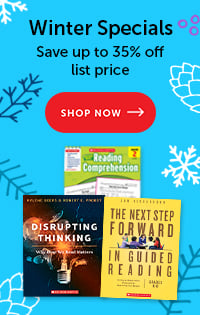The image depicts a promotional section from an online bookstore's webpage, highlighting their "Winter Specials" sale. The offer boasts savings of up to 35% off the list price. Dominating the scene is a prominent red call-to-action button, urging users to "Shop Now" in bold white lettering, accompanied by a rightward arrow. 

The visual appeal is enhanced by a trio of book covers prominently displayed: 

1. **Reading Comprehension**: An educational book aimed at enhancing children's reading skills.
2. **Disrupting Thinking**: A business analysis book that challenges conventional thought processes.
3. **The Next Step Forward in Guided Reading**: An intriguing guide focused on advancing reading instruction techniques.

The backdrop of the promotional section features a light blue color, adorned with whimsical illustrations of snowflakes and pine cones, reinforcing the winter theme in harmony with the "Winter Specials" headline. This seasonal motif, combined with the clearly marked discount and the diverse selection of books, effectively captures the festive, book-loving spirit.